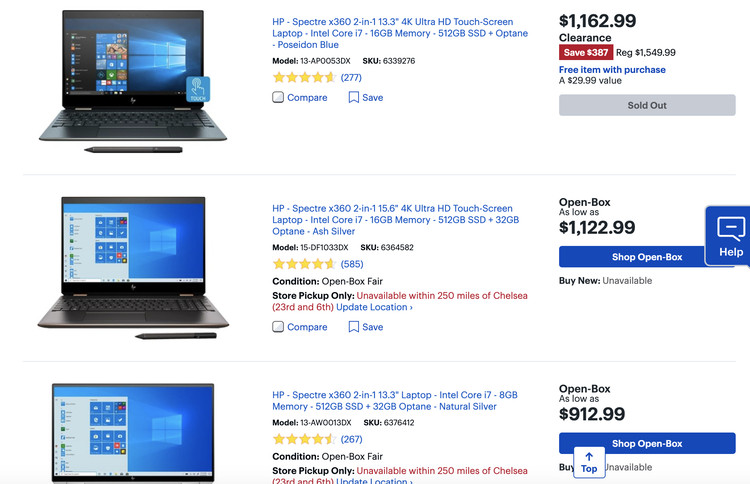This image showcases a comparison of three HP Spectre x360 laptops on an online store webpage. Each laptop features detailed descriptions and pricing:

1. **HP Spectre x360 13.3-inch 2-in-1 Laptop**:
   - **Display**: 10.3-inch 4K Ultra HD touchscreen.
   - **Specifications**: Intel Core i7, 16GB memory, 512GB SSD, plus Optane memory.
   - **Color**: Poseidon Blue.
   - **Rating**: 4.5 stars based on 277 reviews.
   - **Price**: Originally $2,000.99, now on clearance for $1,962.99 (save $277.00).
   - **Availability**: Sold out.
   - **Additional Info**: A button for comparing or saving the item. There is also an indication of a free item with purchase and a direct offer of $1.54.

2. **HP Spectre x360 15.6-inch 2-in-1 Laptop**:
   - **Display**: 15.6-inch 4K Ultra HD touchscreen.
   - **Specifications**: Intel Core i7, 32GB Optane storage.
   - **Condition**: Open box, fair condition.
   - **Availability**: Pickup only, unavailable within 250 miles of Chelsea.
   - **Pricing**: "Open box" price starting at $1,122.99. There is an option to "shop" open box or purchase new, though new is unavailable.

3. **HP Spectre x360 13.3-inch 2-in-1 Laptop**:
   - **Display**: 13.3-inch 4K Ultra HD touchscreen.
   - **Condition**: Open box.
   - **Price**: $1,912.99.

Each listing includes a mix of new, clearance, and open box items, with various availability and pricing options.